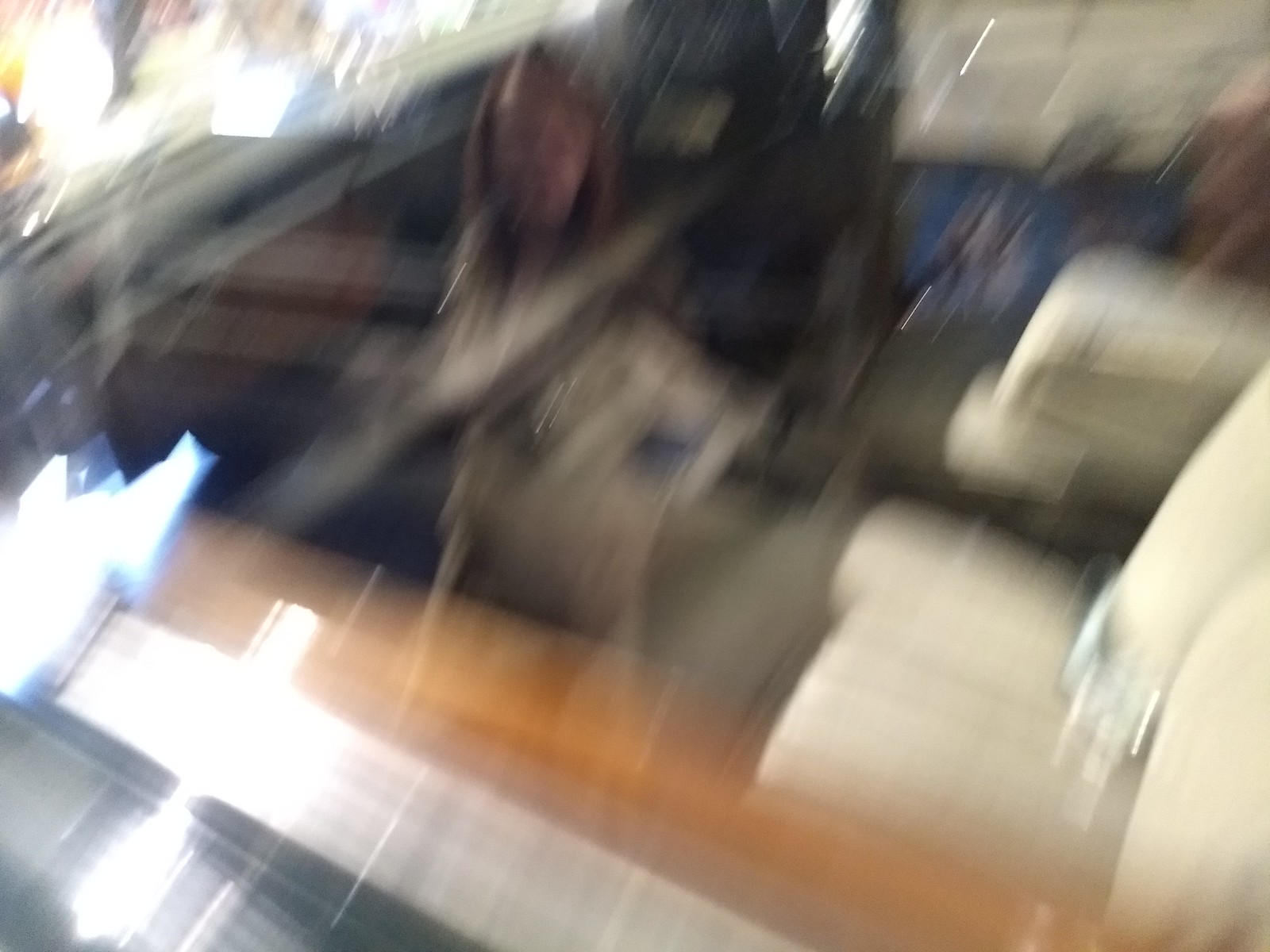This blurry photograph captures the interior of what is likely an RV. The focal point is undefined, but several key details emerge. Visible towards the bottom right is a seatbelt, suggesting the image was taken inside a moving vehicle. The seats, upholstered in a thick tan cloth, further support the RV identification. A wood grain door frame adds a touch of rustic charm, and in the top left corner, a windshield is partially visible, accompanied by a long dashboard below it. Another seat appears faintly in the background on the left, completing the cozy yet cluttered scene.